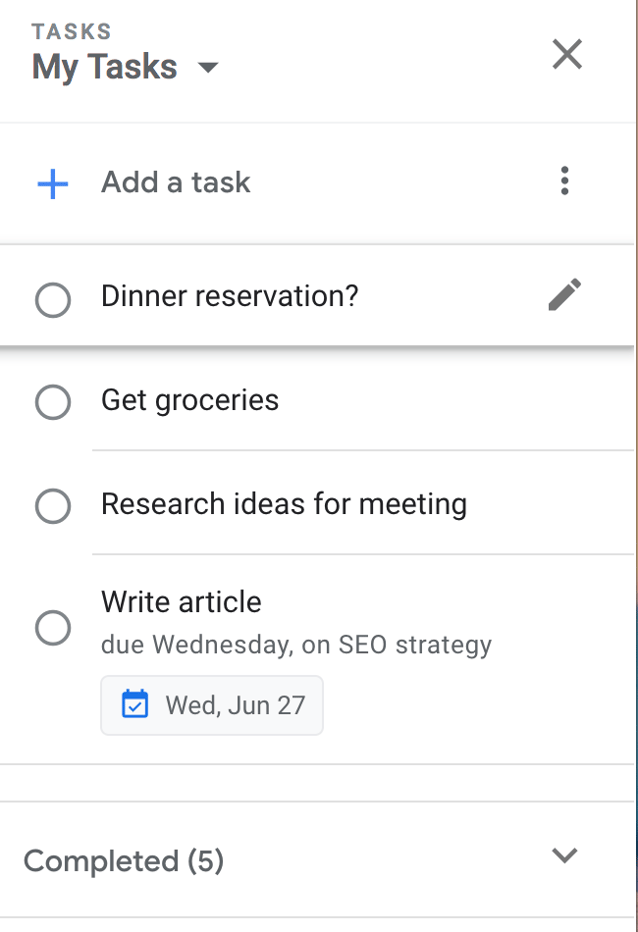Screenshot of a To-Do List App Interface

The screenshot displays a mobile phone interface featuring a to-do list application. The layout is composed of a predominantly white background with black and grey text and various interactive elements.

On the right-hand side of the screen, there is a very thin, dark grey vertical line. At the upper left corner, in lighter grey text, is the abbreviation "TAS". Directly below this label is a button labeled "My TAS" with a dropdown arrow, allowing for modifications. There is also a grey "X" on the right-hand side, presumably for closing or dismissing the view.

Beneath this section is a thin grey horizontal line, followed by a blue checkmark icon. Next to the icon, in black text, it reads "Add a TAS," accompanied by three vertical dots on the right for additional options. 

Moving further down, the interface displays a list of tasks with clickable circles to mark completion. The first task is "Dinner Reservation," which appears bolded with a pencil icon next to it for editing. Below this is the task "Get Groceries," followed by "Research Ideas for Reading," "Write Article," and then "Do SEO on Wednesday," where "SEO" is capitalized. 

Next to the "Do SEO on Wednesday" task, there is a small blue calendar icon with a blue check mark inside it. This is followed by text stating "When: June 27th" to indicate the due date, which falls on a Wednesday.

At the bottom of the list, there is a section labeled "Completed 5" with a dropdown arrow on the right, likely for viewing completed tasks. 

Overall, the interface is designed for easy navigation and task management, with various icons and buttons to facilitate user interaction.